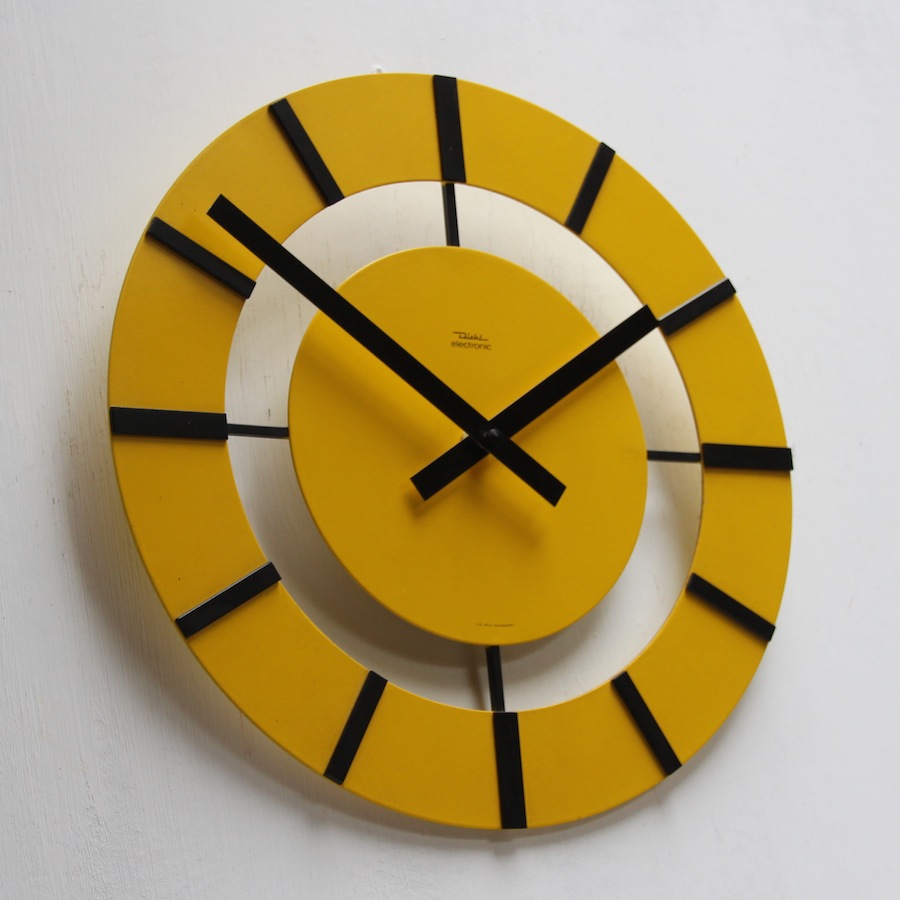The image features a prominently displayed yellow clock against a muted background. The clock is designed with a solid yellow center and an outlined yellow circle surrounding it, creating a distinctive visual appeal. Protruding from its center are two black hands – one shorter for the hour and one longer for the minutes, both indicating a time of approximately 1:52 or 1:57. Surrounding the clock's face are twelve small black rectangles, symbolizing the numbers 1 through 12. A subtle shadow extends behind the clock, enhancing its three-dimensional effect. Notably, the clock is slightly slanted towards the right, adding a dynamic touch to the composition.